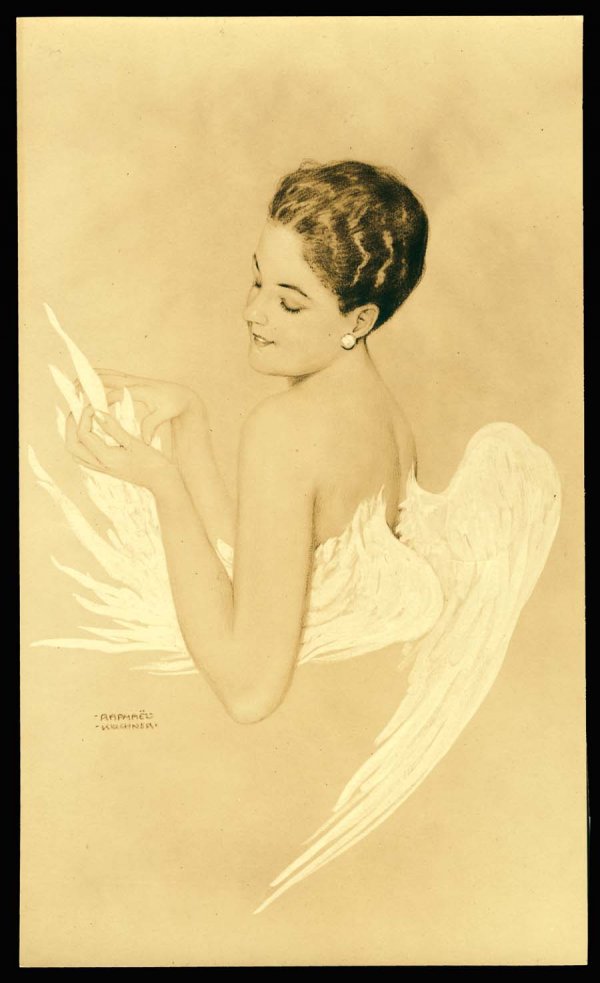The image depicts a detailed painting encased in a black frame. Set against a beige-yellow, almost peachy background that melds with the subject's skin tone, the portrait features a smiling woman with short, brown hair. She wears a prominent round earring and has her head turned slightly, looking downwards. Her eyes appear to be closed, and she is adorned with two large, white angel wings emerging from her back. She gently pets the feathers of the wing under her left arm with both hands, while the other wing droops gracefully to the side. The woman's features, including her neatly trimmed eyebrows and serene expression, are meticulously rendered. There is a signature on the left side of the painting, near one of the wings but not in the corner.